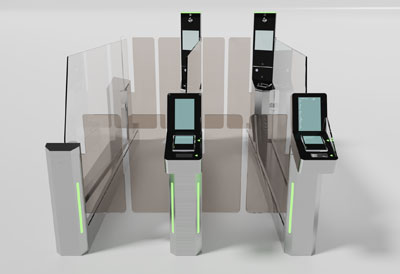The image showcases a sophisticated checkout system, featuring four distinct black scanning devices, each equipped with turquoise screens and green light indicators. The setup includes glass doors or turnstiles designed to open and allow passage once a user checks in or scans a credential. Flanking either side of the scanning stations are translucent glass panels, forming clear lanes for individuals to walk through. The devices, which could also be cameras or volume measuring tools, are positioned atop gray bars—though one bar on the left side is missing a device. The entire system is encased by glass walls extending a few feet high, set against a light gray background, creating a modern and high-tech ambiance.